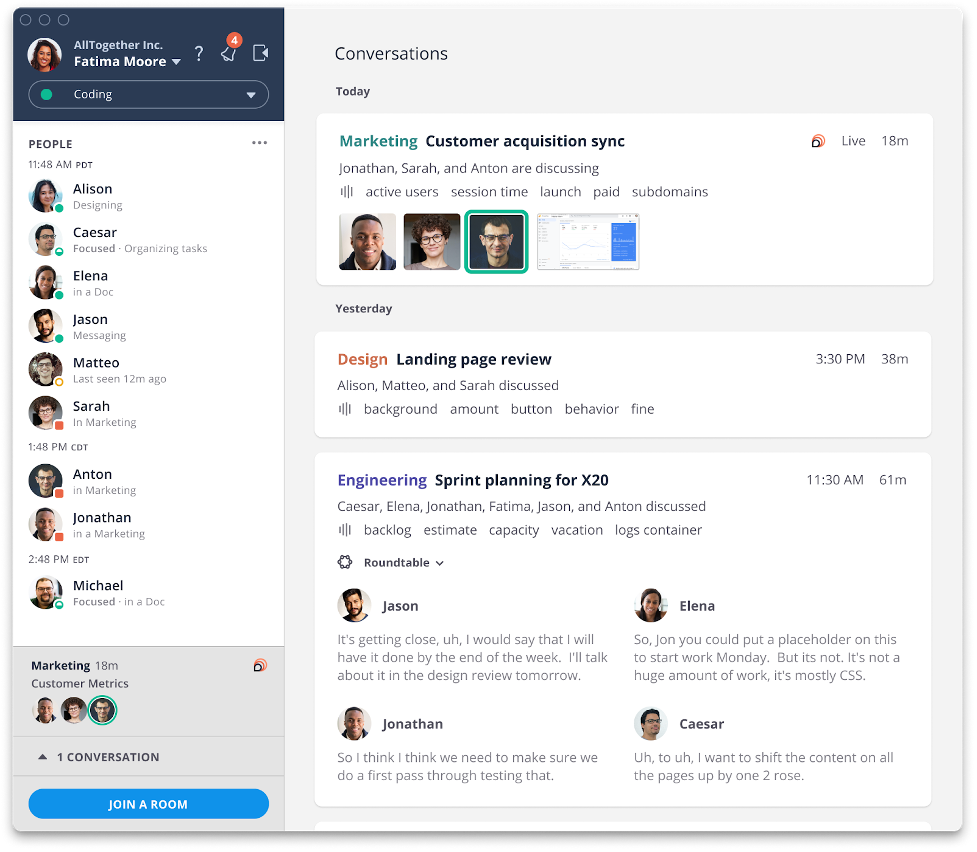**Detailed Caption:**

The screenshot displays an interface of a communications app, likely facilitating open discussions and team collaborations, under the organization "Altogether Inc." At the top left corner, it indicates "Fatima Moore". Below this, a category labeled "Coding" is listed, followed by "People". The timestamp reads 11:48 AM PDT.

In the "People" section, the following activities are noted:
- Allison is engaged in designing.
- Cesar is organizing tasks.
- Elena is working within a document.
- Jason is messaging Mateo, who was last seen 12 minutes ago.
- Sarah is focusing on marketing.

Additionally, at 1:48 PM CDT:
- Anton and Jonathan are both assigned to marketing tasks.

At 2:48 PM EDT:
- Michael is actively working within a document.

Under the "Marketing" section, it states there are "18M customer metrics," along with an indication of "one conversation." There is also a prominent blue button labeled "Join a Room."

On the right side of the interface, the app seems to provide detailed expansions of these various sections, although specific details of this elaboration are not visible in the screenshot.